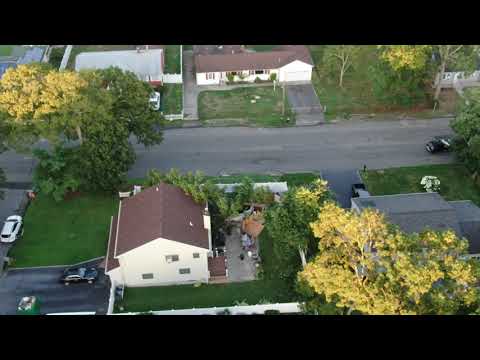This aerial photograph captures a suburban street corner, viewed from above. The composition features a two-lane paved street without any visible markings, flanked by a variety of homes. At the top of the image, three distinct houses are visible amongst abundant greenery. To the left, partially hidden by a large green tree, is the first house. The central home, characterized by its long, narrow structure and single-car garage with a brown roof, stands prominently. The third house in the upper right corner is a quaint, storybook-style home. 

The scene below is equally detailed: on the left side of the street closest to the viewer, a well-maintained square green yard is noticeable. A white car is parked on a side street nearby. A black car is also visible, parked in a driveway in the lower-left corner. The image prominently features a two-story white house with a brown roof, occupying the bottom center. Its spacious backyard includes a stone patio. The lower right corner of the photograph reveals another large tree extending over a grey roof. 

The foliage in the neighborhood showcases various shades of green, transitioning into lighter hues, indicative of seasonal change. The lawns show mixed care, with some neat and trimmed while others appear patchy. The serene neighborhood ambiance is interrupted only by a few parked cars and a single car seen moving along the road.